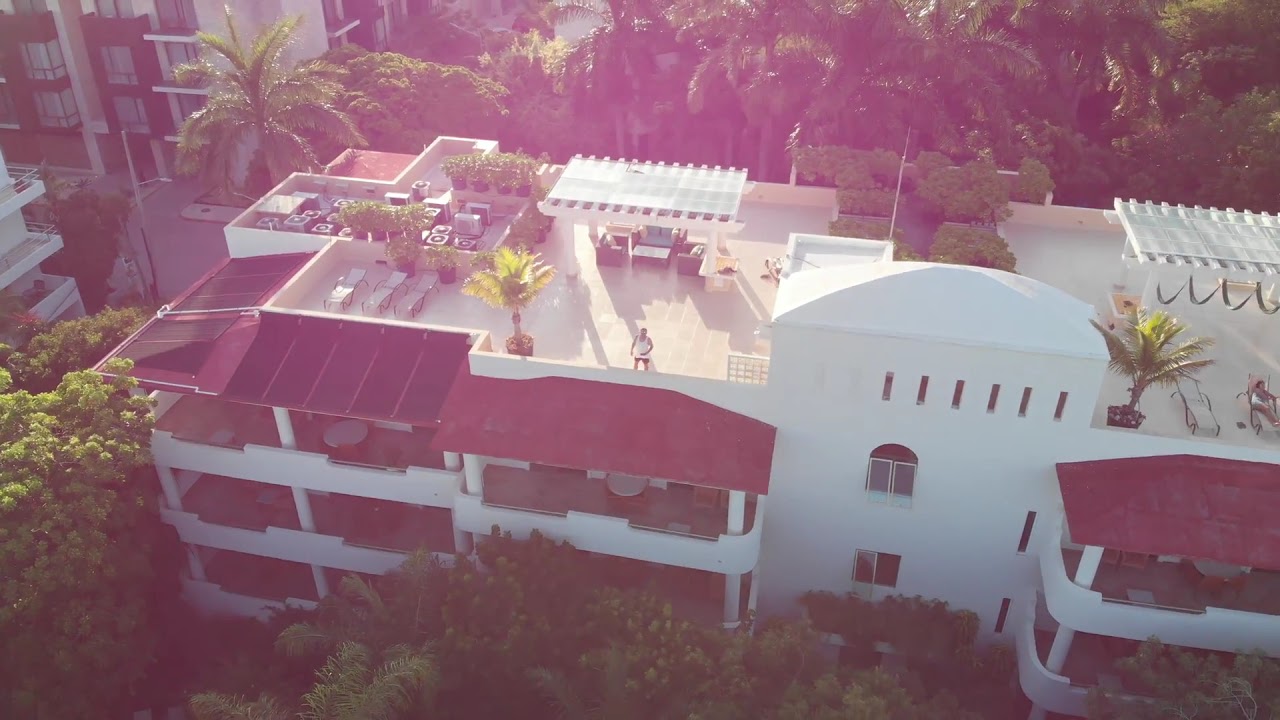This aerial daytime photograph showcases a large, multi-story white building that appears to be a resort or possibly a hotel, standing tall amid a lush array of trees, including numerous palm trees, leafy bushes, and hedges. The building stretches wide and features three distinct levels, each adorned with balconies that are shaded by red roofing material. On top of the flat main roof, there is an inviting seating area complete with tables, chairs, lounge chairs, potted palm trees, and small gazebo structures, creating a charming outdoor space. A man, light-skinned and dressed in a white tank top and dark shorts, is seen standing on this rooftop area, gazing outward. The building is bordered by additional structures to the left, which may serve as more apartments or hotels. The overall scene captures a serene, tropical environment replete with verdant foliage and well-appointed amenities.